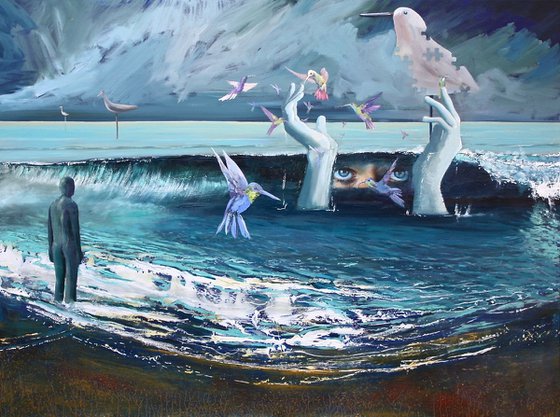In this modern expressionistic painting of a turbulent ocean scene, the foreground features a dark brown beach with waves lapping against its edge. The water showcases various shades of blue and white, capturing the dynamic movement of the waves. On the left side of the drawing, a human figure, sculpted in a dark greenish-blue clay-like material, stands at the water's edge. The figure is seen from behind, appearing virtually naked and gazing into the ocean.

Central to the composition is a wave curling toward the shore, revealing a pair of large, sparkling blue eyes beneath its crest. Emerging from the water, icy blue forearms extend upward, each hand actively interacting with the scene. The right hand holds a vivid pink bird with missing puzzle pieces, adding an air of mystery. Surrounding the scene are multiple hummingbirds, including a prominent blue one hovering over the water in the center, and others scattered throughout the background.

The backdrop is dominated by a stormy, bluish-gray sky, adding to the intensity and drama of the scene. Together, these elements create a powerful, highly detailed tableau of modern artistic expression, imbued with layers of surreal and symbolic imagery.